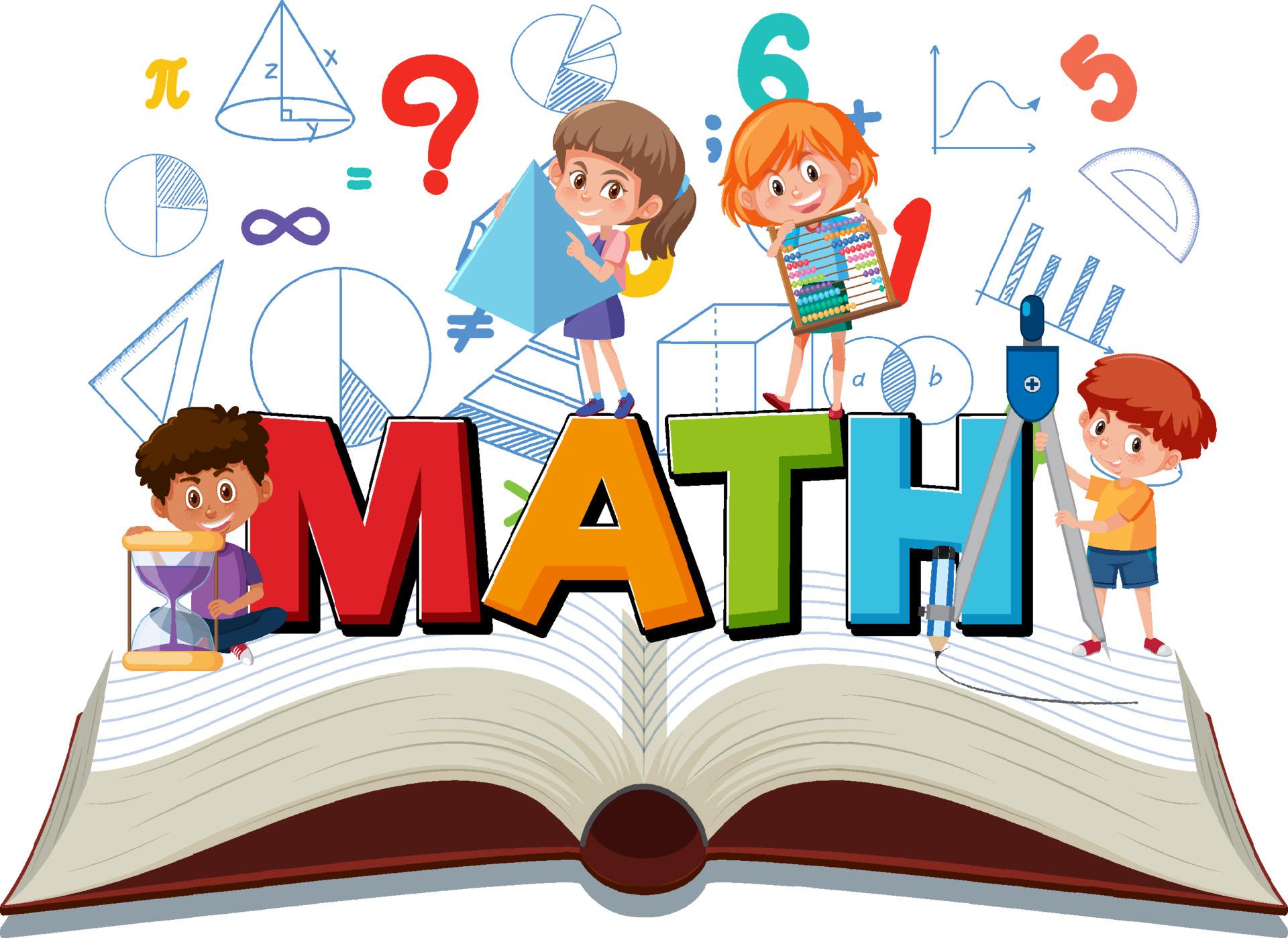The digital artwork features a vibrant and educational scene centered around the theme of "math." At the foreground is an open book with white, blue-lined pages, serving as a platform for the characters and objects. Above the book, the word "MATH" is prominently displayed in large, colorful capital letters—'M' in red, 'A' in orange, 'T' in green, and 'H' in blue.

To the left of the word "MATH" stands a boy with brown hair in a purple shirt, holding an hourglass. On the right side is another boy with red hair, dressed in a yellow shirt and blue shorts, holding a protractor. Sitting on the letters 'A' and 'T' are two girls: the girl on the left with brown hair holding a triangle, and the girl on the right with red hair holding an abacus.

Surrounding this central scene is a background filled with diverse math-related symbols and imagery, such as an infinity sign, pie chart, bar graph, geometric shapes (including cones and spheres), and various numbers. The colors of blue, orange, and yellow add to the bright and clear atmosphere of the image.

Overall, the detailed and lively composition captures the essence of learning and exploring mathematics through a playful and engaging digital illustration.